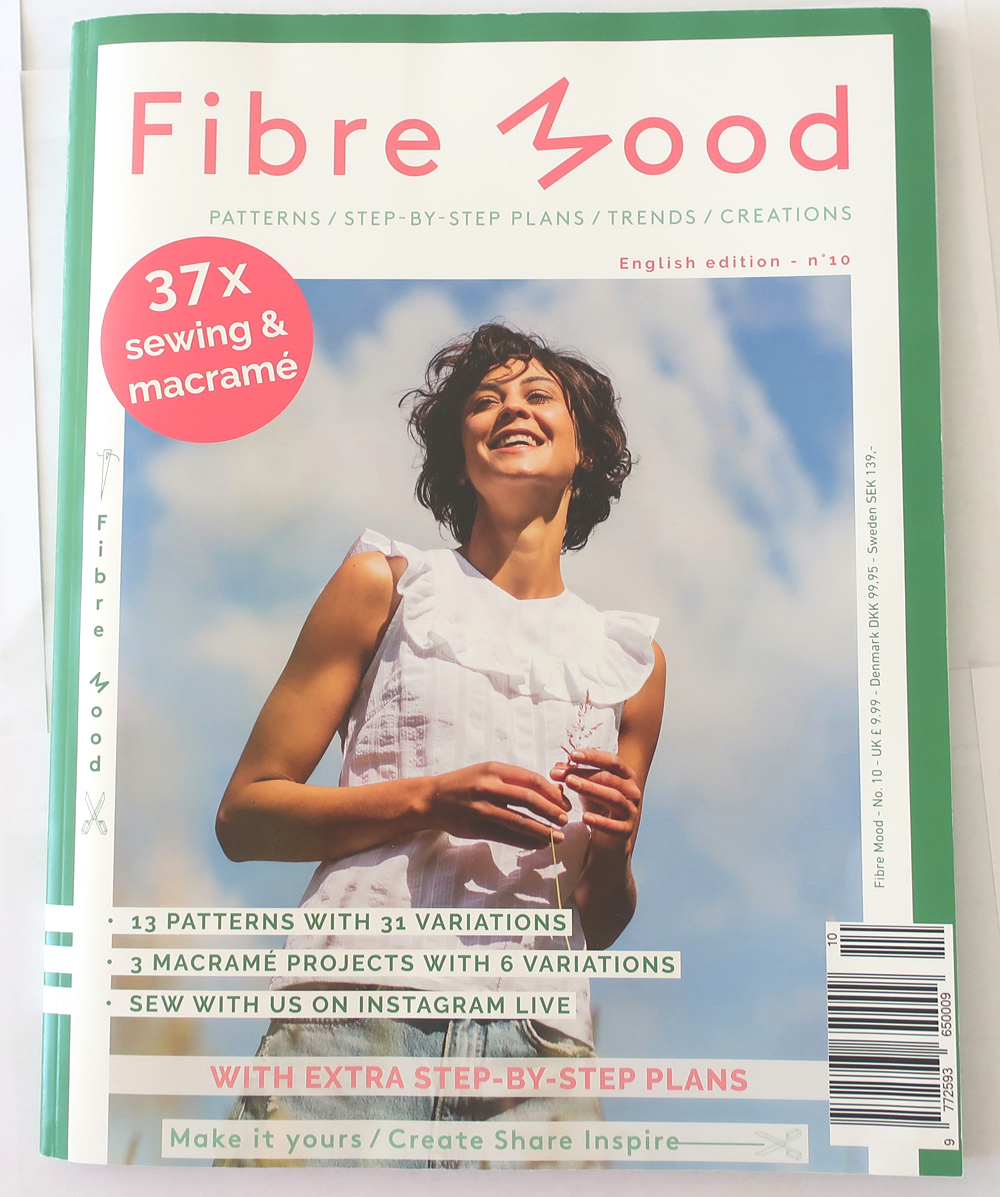The cover of the vertically aligned, rectangular magazine features a green border with a white background. At the top, the title "Fiber Mood" appears in red letters, with the "M" tilted sideways. Below it, in smaller, green all-caps text, are the words "Patterns / Step-by-Step Plans / Trends / Creations." A red circular information bubble on the left side highlights "37X Sewing and Macrame" in white text.

Dominating the center is a large square photograph of a smiling Caucasian woman with short, curly brown hair. She is wearing a white ruffled sleeveless top and denim bottoms, which are cut off at the thighs in the image. The backdrop is a blue and white sky. The woman is holding a small plant in her hands.

In the lower right corner, there is a barcode, and across her waist on the left side, additional text in green lists "13 Patterns with 31 Variations," "3 Macrame Projects with 6 Variations," and "Sew with Us on Instagram Live." Centered at the bottom, red text reads "With Extra Step-by-Step Plans," and further down in green text, the magazine's slogan says, "Make it Yours / Create, Share, Inspire."